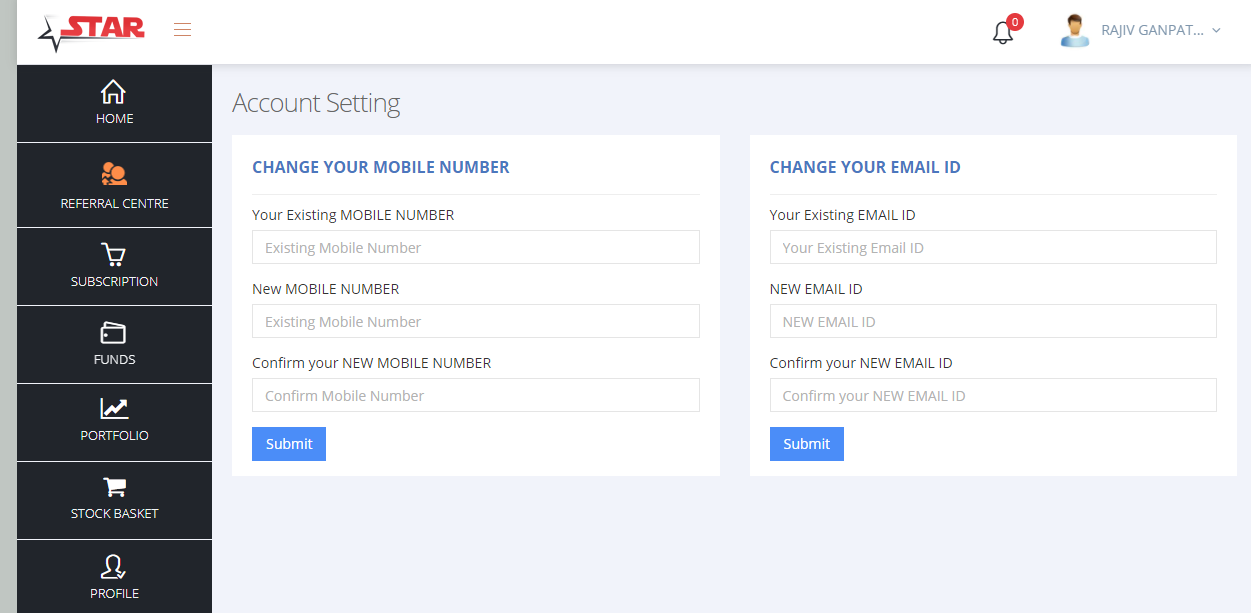This image is a screenshot of the STAR website. In the upper left-hand corner, the word "STAR" is prominently displayed in red, all uppercase letters, with the STAR logo emerging from the letter "S". The site features a vertical menu on the left side of the screen. The menu options listed from top to bottom are: Home, Referral Center, Subscription, Funds, Portfolio, Stock Basket, and Profile.

On the main part of the screenshot, to the right of the vertical menu, the section titled "Account Settings" is visible. This section includes a section labeled "Change Your Mobile Number," which contains text input fields for the existing mobile number, the new mobile number, and the confirmation for the new mobile number. Adjacent to this, there is another section titled "Change Your Email ID," which features text input fields for the existing email address, the new email address, and the confirmation for the new email address.